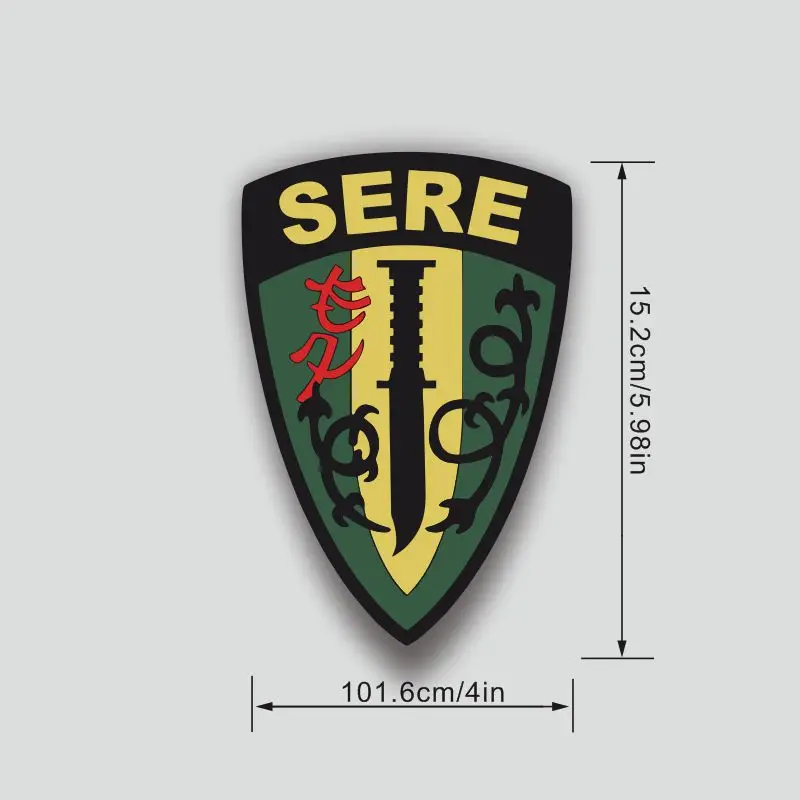This horizontal rectangular photograph features a patch laid on a gray surface, delineated with measurement arrows indicating dimensions of 101.6 centimeters (4 inches) horizontally and 15.2 centimeters (5.98 inches) vertically. The patch resembles a coat of arms shaped like the tip of a knife blade. Dominating the top section is a black arc emblazoned with "S-E-R-E" in large, gold letters. Central to the design is a gold knife blade shape with a black depiction of a downward-curving knife featuring an irregular handle. Flanking the knife are areas of green interspersed with red and black elements, with some of the lettering appearing to be in Japanese. The detailed, ornamental design evokes a sense of military or tactical insignia, poised to be sewn onto a jacket or shirt.